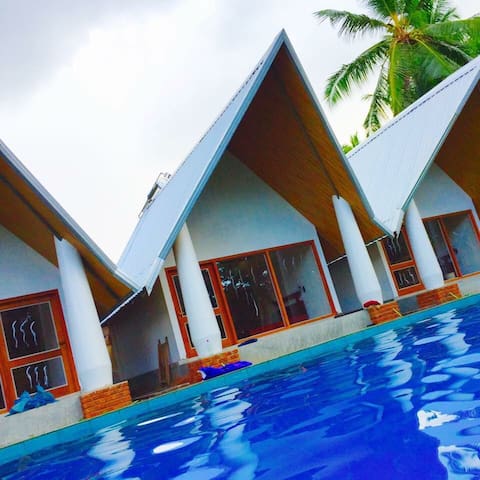The image is an advertisement for a scenic vacation resort featuring charming bungalows arranged diagonally from the bottom left to the top right. Each bungalow, bearing a distinctive pointed, triangle-like roof and held up by white pillars, invites guests with spacious, brown-tinted windows and large doors, potentially doubling as sliding doors. The bungalows, set against a backdrop of a cloudy yet blue sky, exude an inviting charm under the natural light, which seeps through despite the modest cloud cover. Each unit also includes fold-up chairs outside, ideal for leisurely relaxation.

In the foreground, an expansive, sparkling blue pool stretches out, adorned with playful dolphin-shaped lounge floaters, suggesting a fun and relaxing atmosphere. The bungalows are so close to the pool that one might step right from their bedroom into the refreshing water with minimal effort. Adding to the tropical ambiance, a tall, lush palm tree stands prominently in the top right corner of the image, soaring above the bungalows. The pool area itself features a light blue border, enhancing the serene visual appeal of this picturesque resort setting.